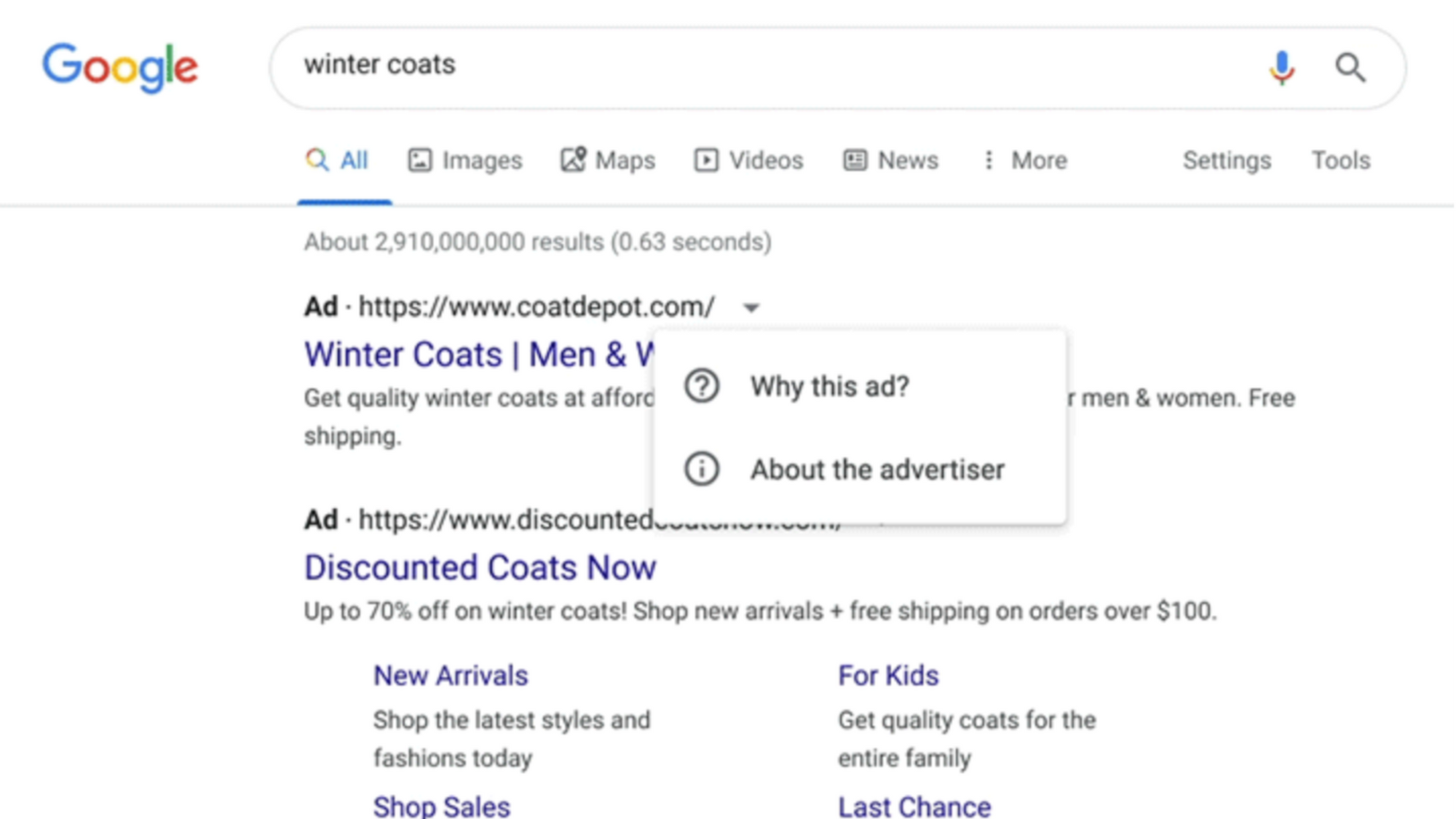This image is a screenshot of a Google search result page for the query "winter coats". In the upper left corner, the Google logo is prominently displayed, followed by the search bar to its right, which includes both a microphone icon and a magnifying glass icon on the far right. The search query "winter coats" is entered into the search bar.

Below the search bar, the interface showcases a menu with various tabs including "All," "Images," "Maps," "Videos," "News," "More," "Settings," and "Tools". Beneath this menu, the search duration data is displayed, indicating how long it took to generate the results.

The first result is a sponsored ad from https://www.coatedepot.com, accompanied by pop-up boxes labeled "Why this ad?" and "About the advertiser". The second sponsored ad promotes discount coats, offering up to 70% off on winter coats, highlighting new arrivals, and noting free shipping on orders over $100.

Further down, several clickable categories are displayed in blue buttons: "New Arrivals for Kids," "Shop Sales," and a prominent "Last Chance" button in red.